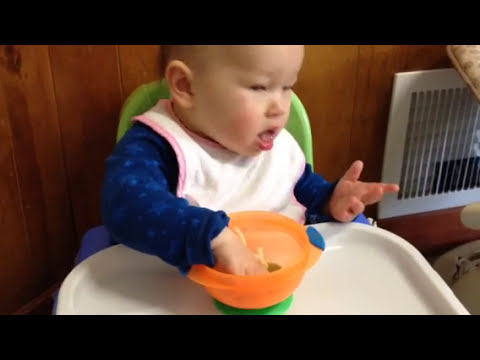The image captures an infant seated in a green high chair with a blue table in front. The baby, appearing to be of light skin complexion, possibly Asian, is wearing a white bib trimmed in pink and a blue outfit adorned with light blue stars. With a slightly open mouth and gaze directed to the right, the baby looks engaged and possibly trying to speak. In front of the infant sits an orange cup with blue handles and a green base, containing an indistinct type of food, which the baby is reaching into with its hand. The backdrop is an older-style wood-paneled wall with a white heat vent visible on the right. The image is well-lit, suggesting the lights are on, and framed by black horizontal bars at the top and bottom. The scene is vividly detailed, capturing a bright moment of the baby exploring its food in a colorful, familial environment.